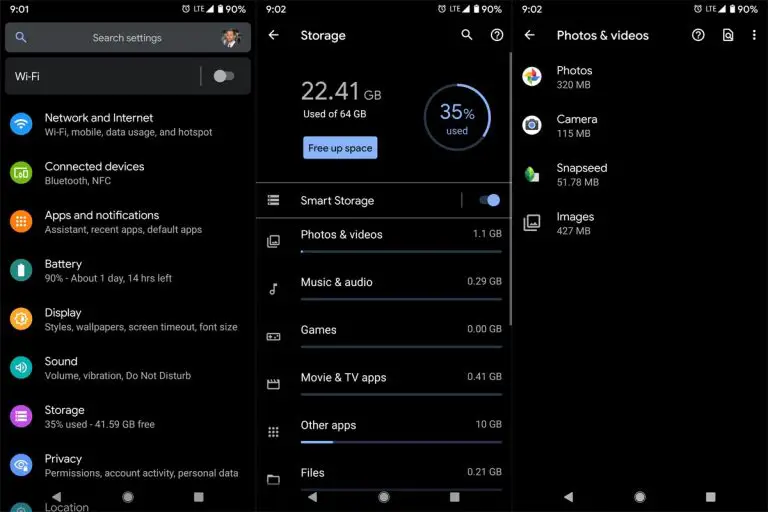The image consists of three vertically aligned screenshots taken from a cell phone. Each screenshot captures different settings pages, arranged in chronological order from 9:01 AM to 9:02 AM.

- **Left Screenshot (9:01 AM)**: This screenshot displays the main settings menu of a smartphone. At the top, there are icons for notifications and other system statuses. Below the header, a search settings bar is visible along with a profile icon. The list below includes various settings options such as:
  - **Network & Internet**: Settings related to connectivity.
  - **Connected Devices**: Options for pairing with other devices.
  - **Apps & Notifications**: Manage app settings and notifications.
  - **Battery**: Information and settings regarding battery use.
  - **Display**: Options to customize the screen.
  - **Sound**: Audio settings for the device.
  - **Storage**: Shows amount of storage used and available.
  - **Privacy**: Settings to manage personal data security.

- **Middle Screenshot (9:02 AM)**: This image focuses on the storage settings. It shows the total storage capacity and the amount currently used. Below this are detailed categories of storage usage, including:
  - **Smart Storage**
  - **Photos and Videos**
  - **Music and Audio**
  - **Games**
  - **Movies and TV**
  - **Apps**
  - **Other Apps and Files**
  Each category lists the amount of space consumed.

- **Right Screenshot (9:02 AM)**: This screenshot delves deeper into the "Photos and Videos" section. It shows usage divided into:
  - **Photos**: General photo storage.
  - **Camera**: Space used by camera images.
  - **Snapseed**: Space occupied by edited images through Snapseed.
  - **Images**: Other image files on the device.

Overall, the image comprehensively captures the user's journey from the main settings menu to specific storage details and focuses on the categories within storage used by photos and videos.